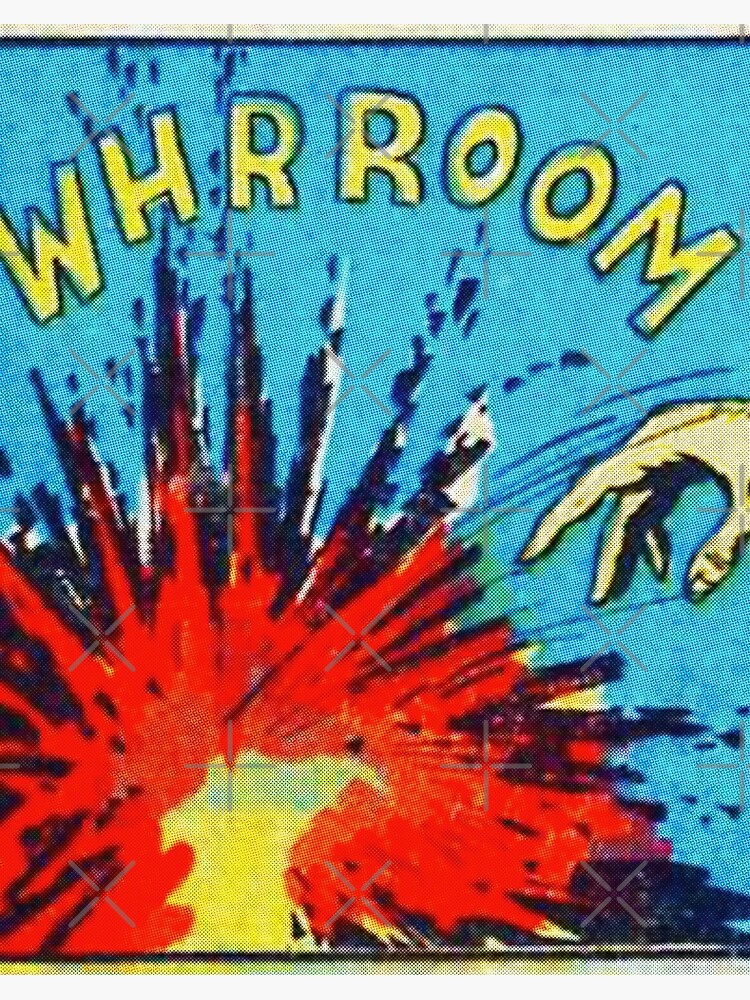This image captures a vivid comic book poster featuring a dynamic explosion. At the bottom left, the explosion's core radiates a vibrant yellow, encircled by intense red bursts that transition to darker shades. To the right, a pale hand, possibly the source of the explosion, extends into the scene, accentuated by motion lines that suggest thrown action. Above, the word "VROOM" stands out in bold, capital yellow letters with a black border. The backdrop of the poster is predominantly blue, with scattered plus sign symbols creating a watermark effect. The entire image has a grainy, papery texture, reminiscent of a classic comic panel.